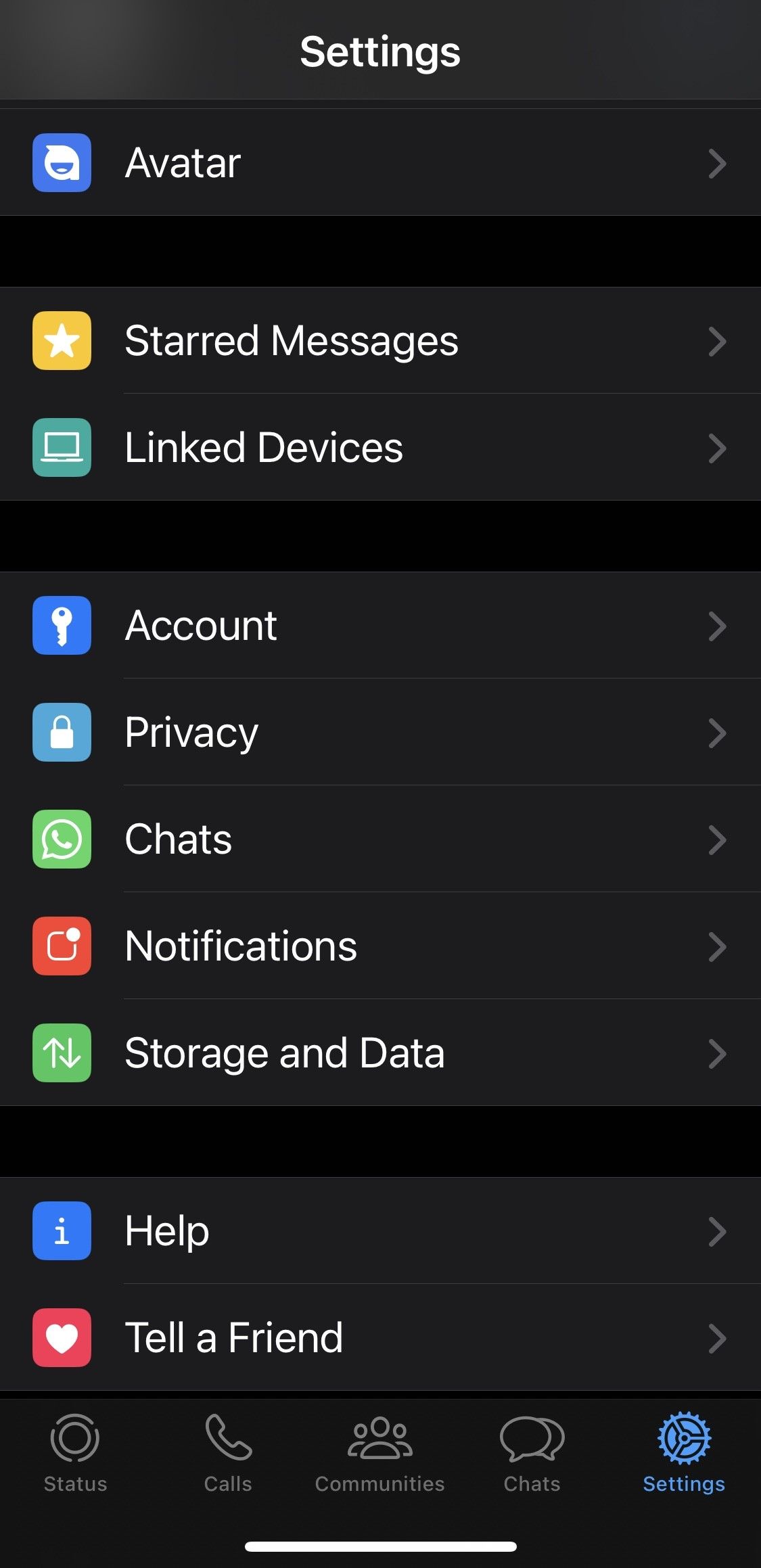The image depicts the settings section of a mobile application. At the top, the title "Settings" is displayed in white text against a dark gray background. Below that is a dark black area with the label "Avatar" in white, accompanied by a small blue square featuring a white alien-like icon.

Next, a dark black section precedes a dark gray area labeled "Starred Messages," highlighted with a gold box containing a white star. Following this is another dark black section leading to "Linked Devices," marked by a green box with an outline of a computer and a connecting line, all in white.

In continuation, another jet black area is followed by a dark gray section listing five options: "Account," "Privacy," "Chats," "Notifications," and "Storage and Data." Each option has a small gray arrow on the far right, indicating it is clickable. Next to "Account" is a blue box with a white key. "Privacy" is represented by a turquoise box with a white lock. "Chats" is illustrated by a green square with a white chat bubble and telephone icon. "Notifications" is marked by a red square containing a white dot. "Storage and Data" features a green square with a white upward and downward arrow.

At the bottom, the image showcases two more options: "Help," indicated by a blue square with a small white "i," and "Tell a Friend," marked with a red square containing a white filled heart icon.

At the very bottom of the image, a menu displays options labeled "Status," "Calls," "Communities," "Chats," and "Settings." These are in gray text except for "Settings," which is highlighted in blue along with a blue settings icon. "Chats" is represented by two small chat icons in gray, "Communities" by three small people icons, "Calls" by an outline of a phone, and "Status" by a design of two circles within a circle.